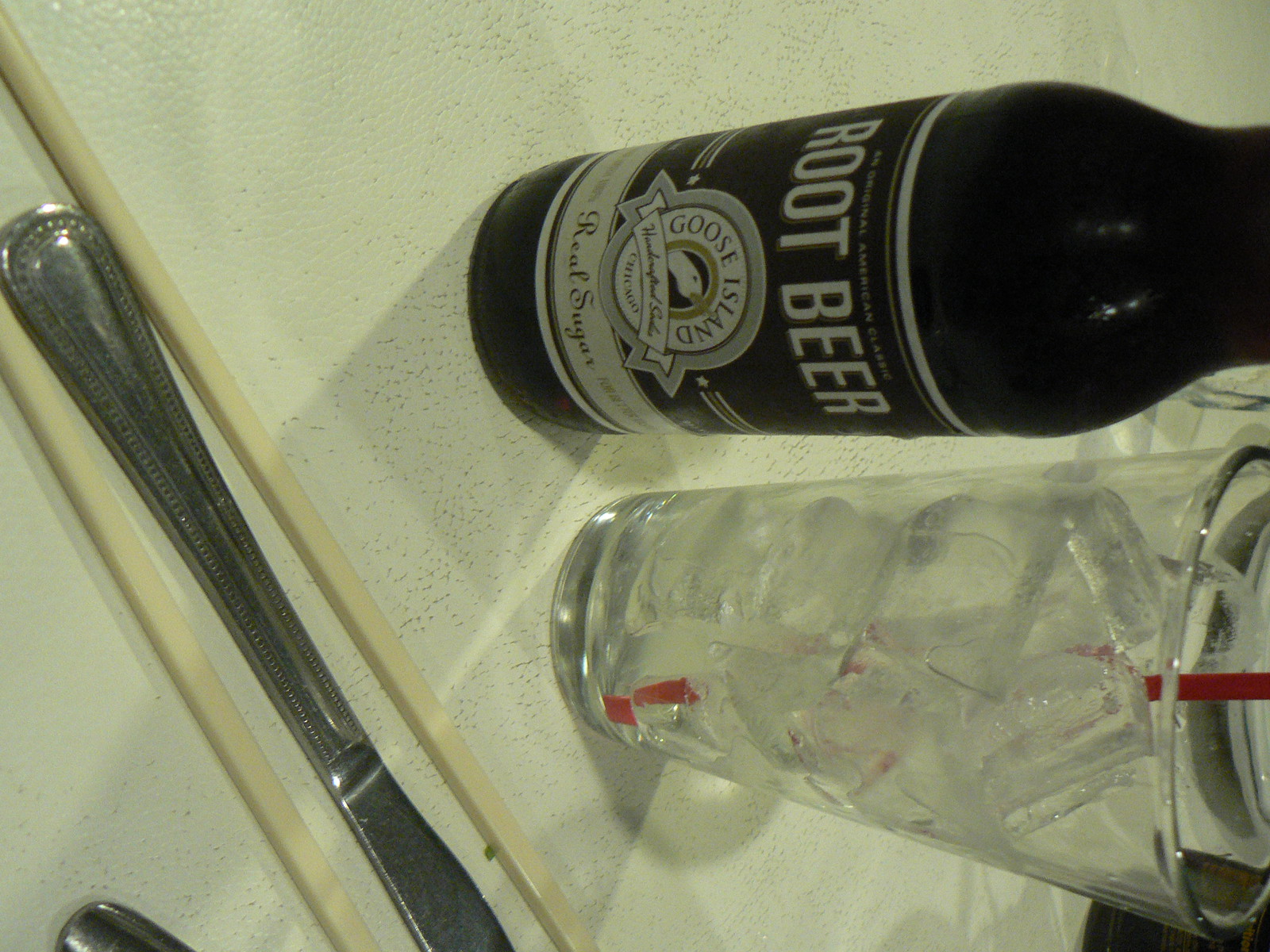This indoor photograph features a close-up of a dark brown Goose Island Root Beer bottle with a black and white label indicating "Root Beer" and "Real Sugar." The label's prominent round logo showcases a goose's head encircled by the words "Goose Island." Adjacent to the bottle on the right is a clear glass packed with ice and a red straw, devoid of any liquid. These items rest on a distinctively white table marred by deliberate textures and pits, filled with noticeable brown grime. In the lower left corner, tan plastic chopsticks and a silver butter knife with a dull edge are neatly placed, with the knife nestled between the chopsticks. Part of another silver utensil is barely visible in the lower right corner of the frame. The overall orientation of the image suggests it might have been taken at an angle or sideways, presenting a detailed snapshot of the table's contents from an overhead perspective.